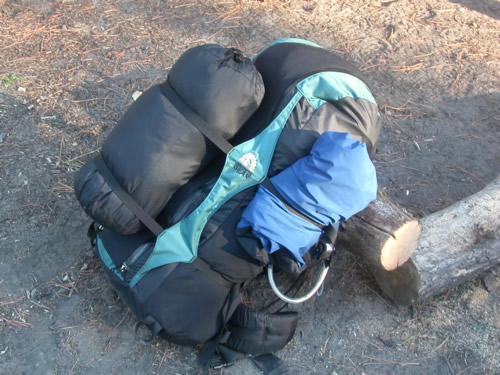This outdoor color photo captures a well-prepared backpacking setup, featuring a large, fully loaded hiking backpack. The black backpack has a striking turquoise stripe and gray accents, and it rests propped against a freshly-cut log, which itself is supported by an older, weathered log. The ground beneath is a sandy clay surface, scattered with small twigs and leaves. The backpack is equipped with various essential items, including a black sleeping bag tightly secured with elastic straps and a bungee cord. A blue hydration bladder is visible, attached to the side with a hose extending to one of the straps for easy access. The backpack casts a shadow to the bottom right, adding depth to the scene. Overall, the photo displays a meticulously organized pack, ready for a rugged hiking adventure.